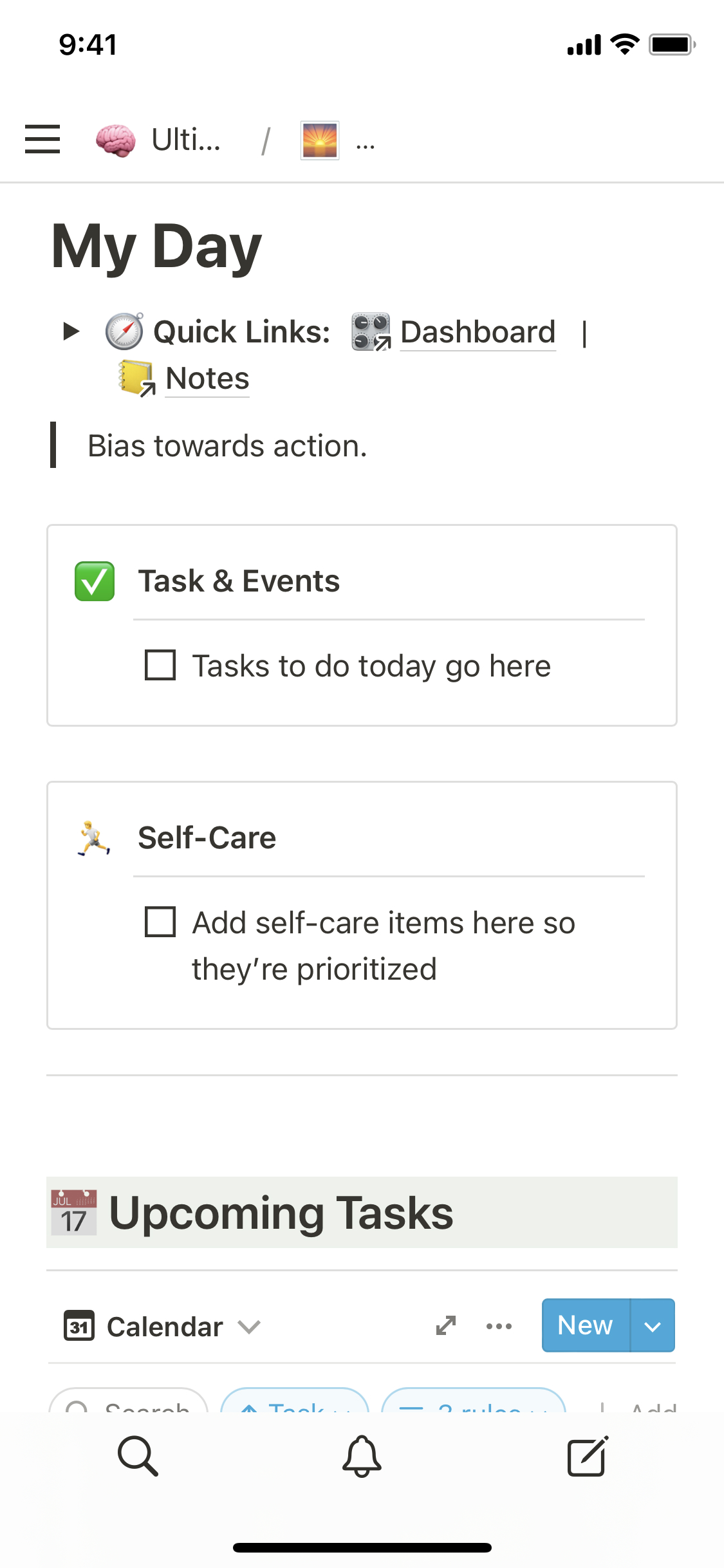The image is a vertical screenshot captured from a smartphone, likely an iPhone, with a white background that appears to be borrowed from a computer screen. At the top left, "9:41" is displayed in bold black text. On the top right, there are icons indicating full signal strength, a Wi-Fi connection, and a full battery.

On the top left again, three horizontal bars are visible next to a small pink icon, followed by the text "ULTI..." and an image of what resembles a sunset. This section is divided by a thin gray line. Below this, in bold black text, it says "My Day," along with several icons for quick links, including Dashboard, Notes, and Bias Towards Action.

Further down, there is a rectangular box labeled "Tasks and Events" featuring a green square with a white checkmark. Below it, placeholder text indicates that tasks to be done today should be added here, next to an empty checkbox.

An icon of a person running is beside the label "Self-Care," reminding users to add self-care items for prioritization. A small calendar icon signifies a section for upcoming tasks, highlighted with bold black text.

Additionally, there are calendar icons, a downward arrow, and an option to "Click on New." The screen is cut off, indicating more content below this section. At the very bottom, navigation icons can be seen above a thick, small black line.